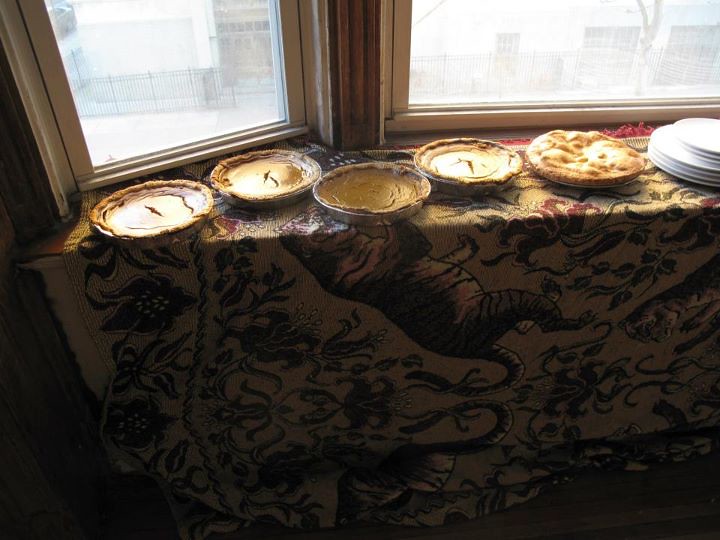This is a color photograph depicting a sunny daytime scene of five homemade pies cooling on a windowsill. The windowsill is covered with a vibrant cloth featuring a mix of floral and animal patterns, including a large tiger and a cheetah. The pies vary in appearance; four look like pumpkin pies with cracked and slightly burnt tops, while the fifth pie, a cream pie with a golden, well-done crust, appears more appetizing. Sunlight filters through the frosted windows, casting shadows and illuminating the scene. Beside the pies, on the right side of the image, is a stack of white plates, consisting of four dinner plates and two or three smaller ones. In the background, visible through the slightly opaque windows, are various buildings, hinting at a business district beyond.